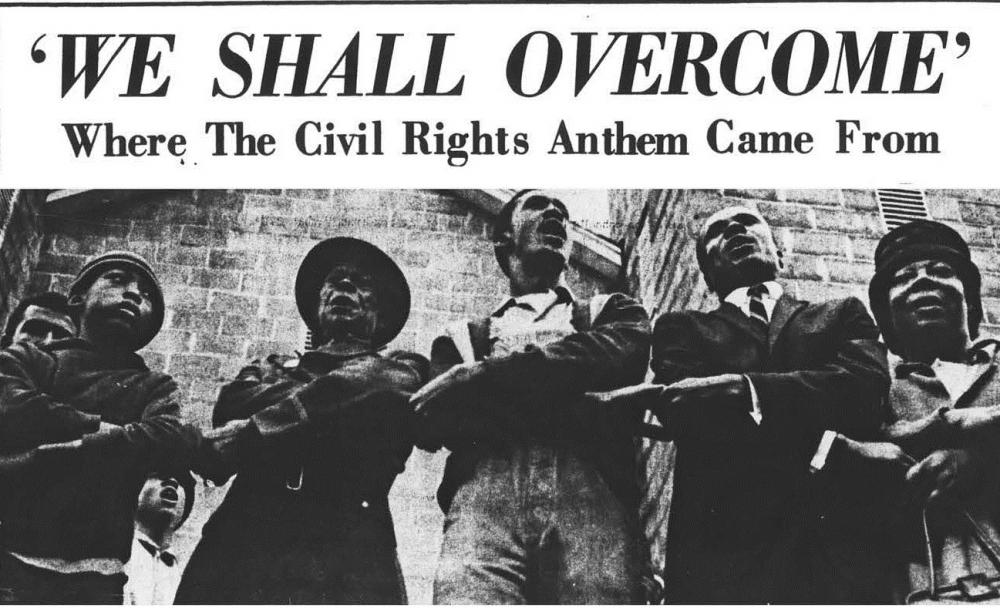This vintage black-and-white image, possibly from a newspaper, features a prominent headline in bold black font that reads, "We Shall Overcome," with the subtitle, "Where the Civil Rights Anthem Came From." The photograph below the heading showcases a group of African American individuals standing in front of a brick building. Taken from a low angle, the image captures seven people, including a child on the left. The group appears to be either singing or speaking, possibly in unison, while holding each other's hands in a crossed manner. Among them are notable figures: a woman wearing a white brimmed hat, a man in overalls and a jacket, a man in a suit and tie, and a woman who seems to be holding a top hat and a cane. The powerful visual emphasizes a sense of solidarity and collective determination, resonating with the Civil Rights movement.